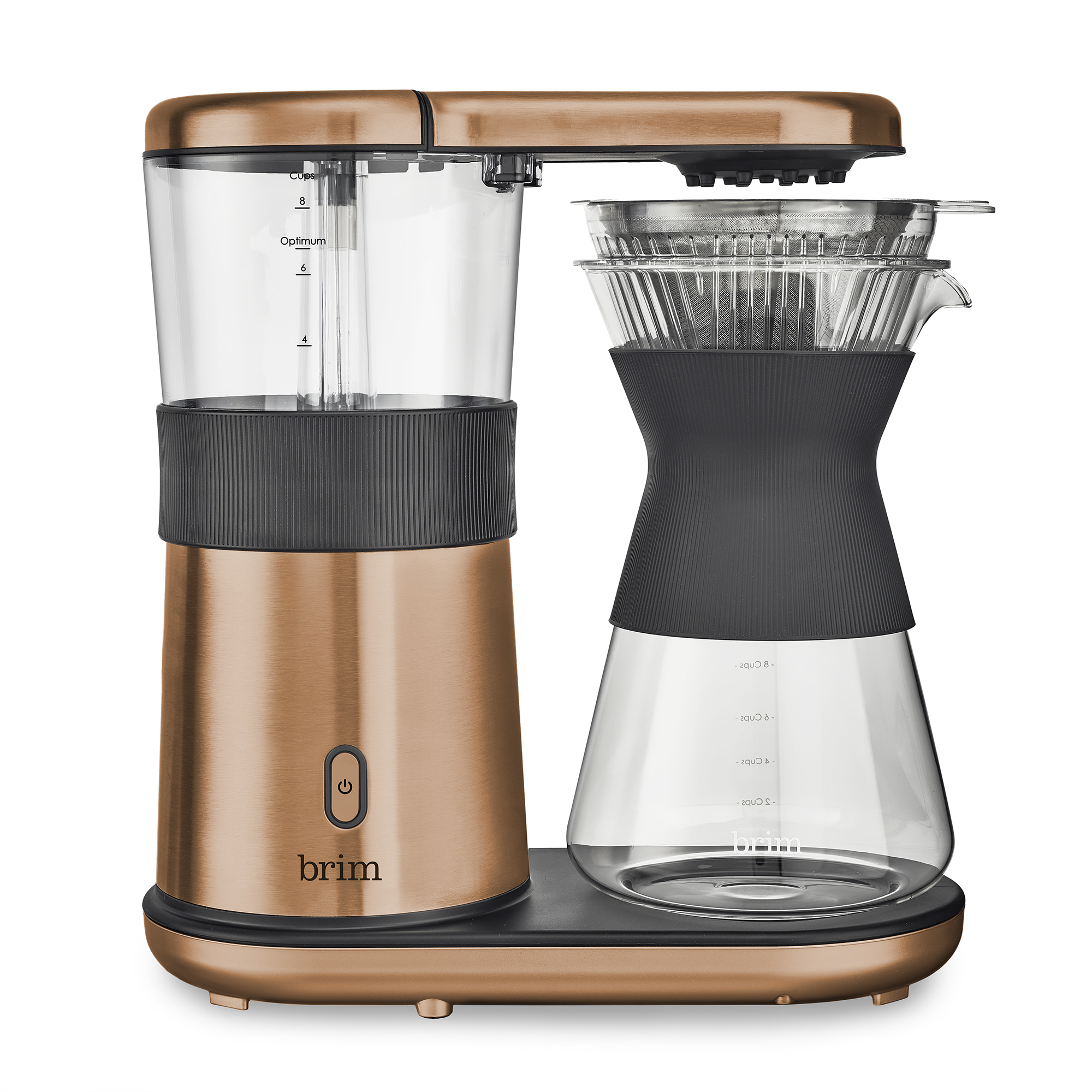This is a detailed product photo of a sophisticated pour-over coffee maker, featuring a stylish bronze color. The coffee maker, branded with the name "Brim" in lowercase black letters located on the bottom left, stands out against its transparent background, giving it an appealing advertising quality. The machine consists of two main sections: a small, clear water tank positioned at the top left, which includes an oval power button, and a sleek glass carafe on the right with a protective black center grip to prevent burns. Notably, the carafe resembles an hourglass and includes measurement markers. The coffee maker is supported by an oval-shaped base that is black on top and bronze at the bottom, complete with small feet for stability.